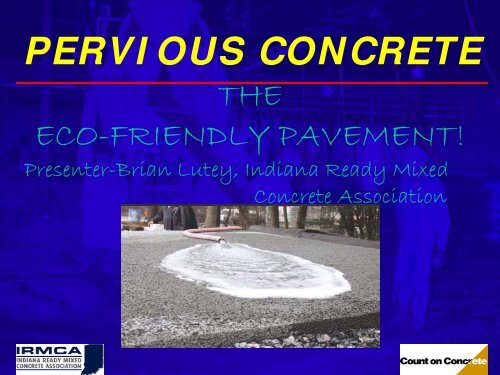The advertisement for the Indiana Ready Mixed Concrete Association showcases their eco-friendly concrete work. At the top, bold yellow letters spell out "Pervious Concrete," underlined by a red line. Below, in blue, slightly frilly font, it reads: "The Eco-Friendly Pavement." Further down, in the same font but smaller, it states: "Presenter, Brian Lutie, Indiana Ready Mixed Concrete Association." The central image depicts concrete being poured through a long tube onto a prepared, gray-framed area, notably surrounded by gravel and a backdrop of trees, though the tops are cropped. The whitish concrete is seen flowing out, covering about a third of the area. At the slide's bottom right, a small label says "Count on Concrete," while the left corner reads "IRMCA, Indiana Ready Mixed Concrete Association." The slide's background is a vibrant variegated blue, giving it a polished and professional appearance.